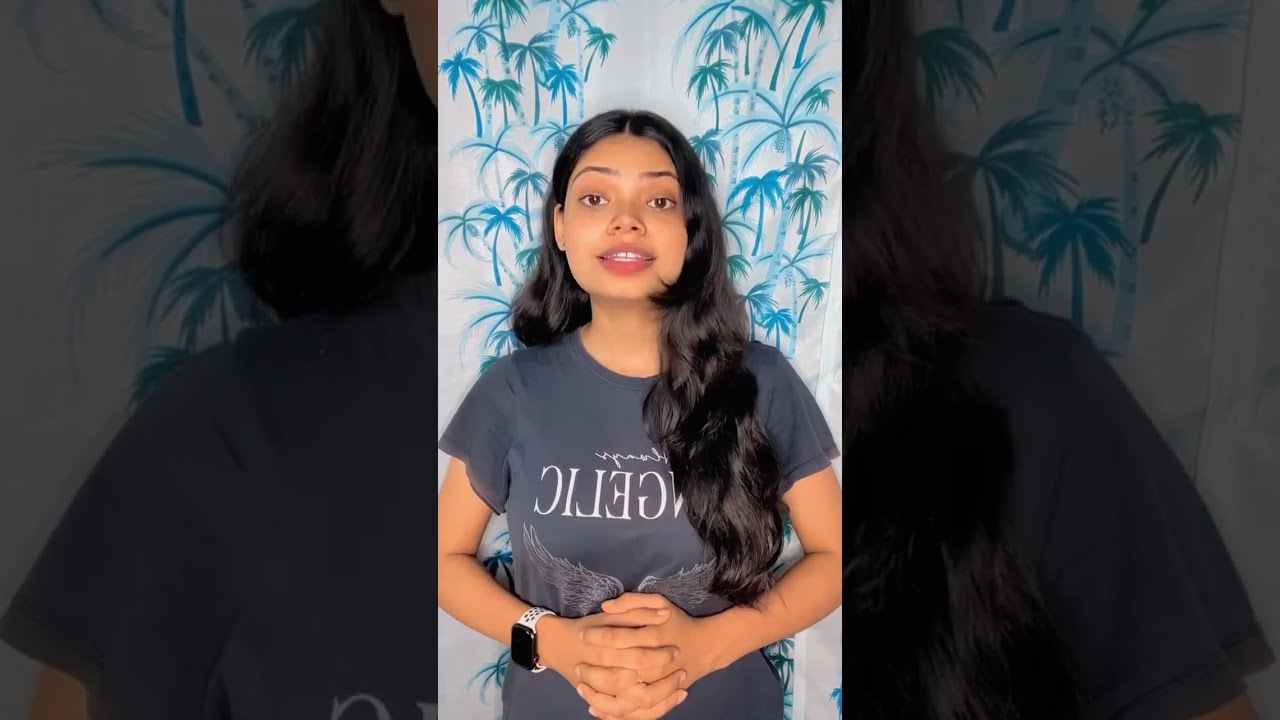In the image, a young woman in her early 20s, likely of Eastern Indian descent, stands poised and staring directly into the camera with a focused expression. Her long, shiny black hair flows down to her waist, partially covering the graphic on her dark gray, short-sleeved t-shirt. The t-shirt features white text and an image of bird wings below the font. On her right wrist, she wears a smart watch with a white band and a black face. She stands with her fingers interlocked in front of her stomach. The background consists of a light blue, white, and lavender wallpaper adorned with blue and green palm trees. The scene suggests she might be engaging in a live stream, interview, or some form of presentation.